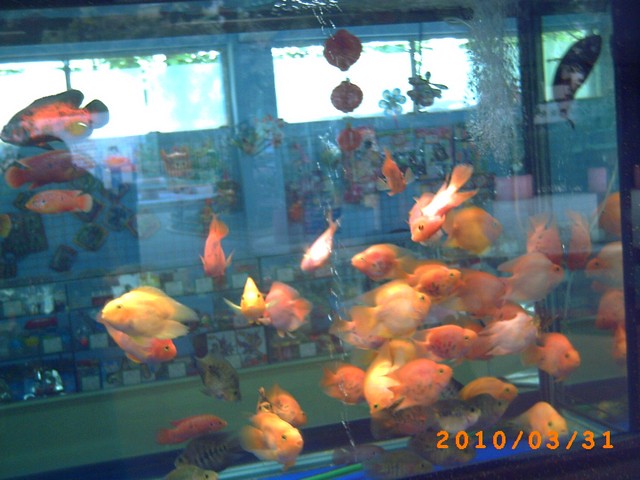This indoor color photograph captures a large, glass fish tank teeming with approximately 30 to 40 oversized, orange goldfish swimming in various directions. The image appears to be taken from outside the aquarium, looking in. In the background, through the clear fish tank, you can see a four-layered red Chinese lantern hanging from the ceiling and windows on the far wall letting in bright light, suggesting it is daytime. The surroundings are somewhat indistinct, hinting at a shop or restaurant setting. Notably, in the bottom right-hand corner of the image, there's an orange date stamp reading "2010-03-31." Additionally, a faint silhouette of the photographer holding the camera up to their face is visible, reflected on the left side of the tank.